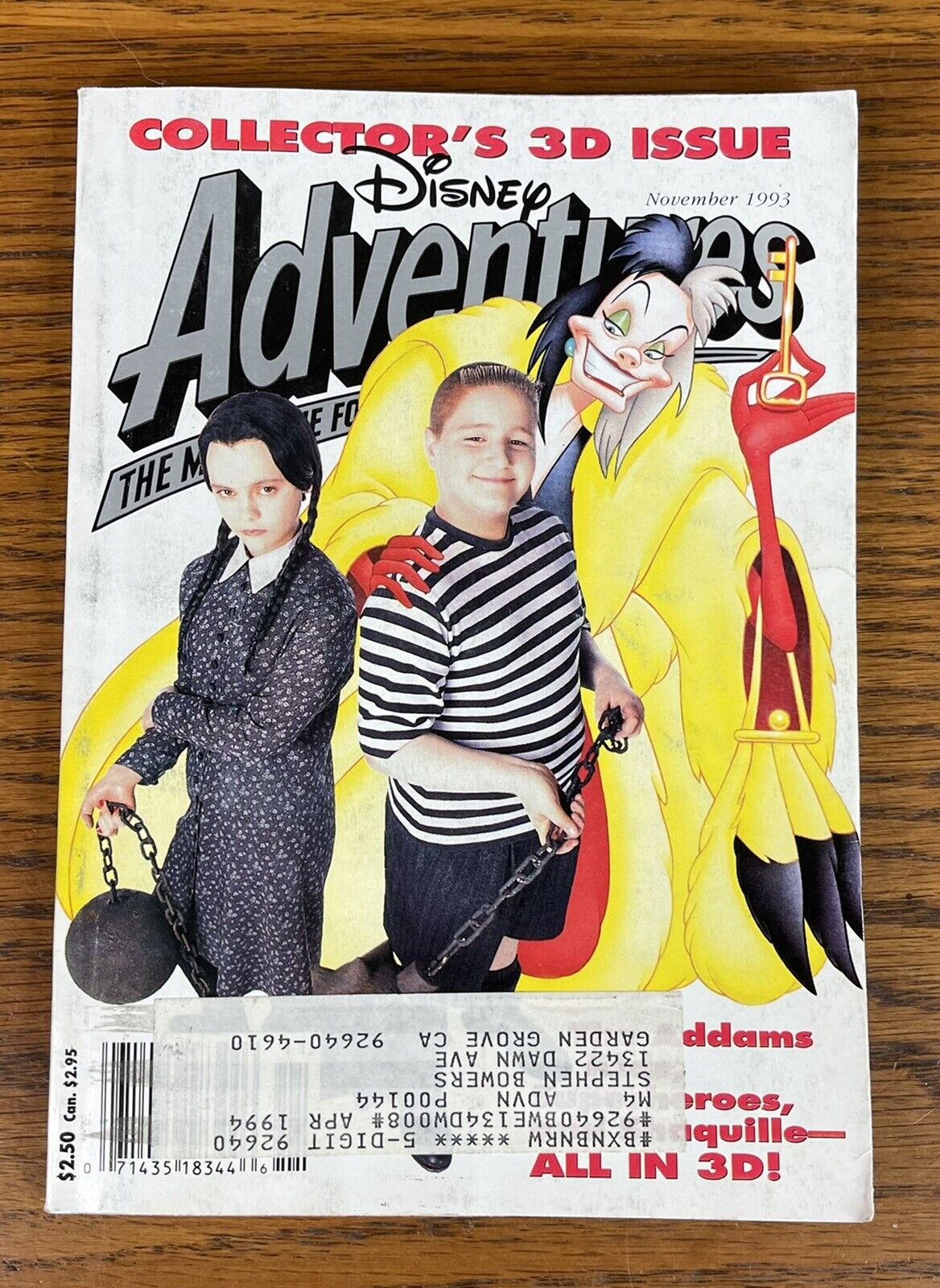This image features a vividly detailed cover of a collector's magazine, captured from an overhead angle, lying on a dark brown, wood-grained surface. The magazine cover, which has a predominantly white background, is well-centered in the photograph with the wood surface visible around its edges. 

At the top, in striking red letters, the text reads: "Collector's 3D Issue." Beneath that, the black Disney logo is prominently displayed, followed by the bold, gray, italicized word "Adventures," highlighted heavily in black. A faint gray band with unreadable black text runs underneath, partially obscured by the characters on the cover.

Dominating the foreground are three iconic characters. To the left, Wednesday Addams from the Addams Family movies stands with her braided pigtails draped over her chest, wearing a gray dress with a white collar. She grips a heavy metal ball and chain in her right hand, gazing intently at the viewer. Beside her is Pugsley Addams, also from the Addams Family movies. He is dressed in a black and white horizontally striped t-shirt, holding the chain with both hands and smiling confidently.

Behind and to the right of the children is a cartoon depiction of Cruella DeVille from Disney's 101 Dalmatians. She is shown in a broad grin, donning a yellow fur coat with black tips and exhibiting her characteristic half-black, half-white hair. In her left hand, she holds a cigarette in a long holder, her red glove complementing her devious expression.

At the very bottom of the cover, an upside-down postal address label partially conceals some red text. However, the words "All in 3D!" in bold red letters are visible in the lower right corner. This detailed depiction highlights the vivid and nostalgic elements of a vintage collector's magazine, dated April 1994.